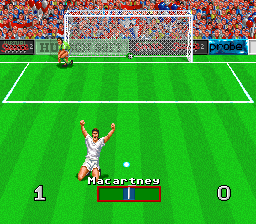The image captures a retro-style video game representation of a soccer game, reminiscent of the classic Gameboy aesthetic. The scene focuses on a soccer field, complete with a goal net and vertical striped lines of alternating light and dark green shades. In the foreground, a player, likely named McCarty, is seen celebrating a recent goal. He is positioned kneeling with his arms triumphantly raised towards the camera, clad entirely in white. The scoreboard on the left side reads '1' while the right side displays '0', indicating that McCarty's team has scored. Behind the goal, digital spectators fill the stands, adding to the atmosphere. To the right, the goalie, dressed in orange, can be seen, likely lamenting the recent score. This moment epitomizes the excitement and intensity of scoring a goal in a classic soccer video game.